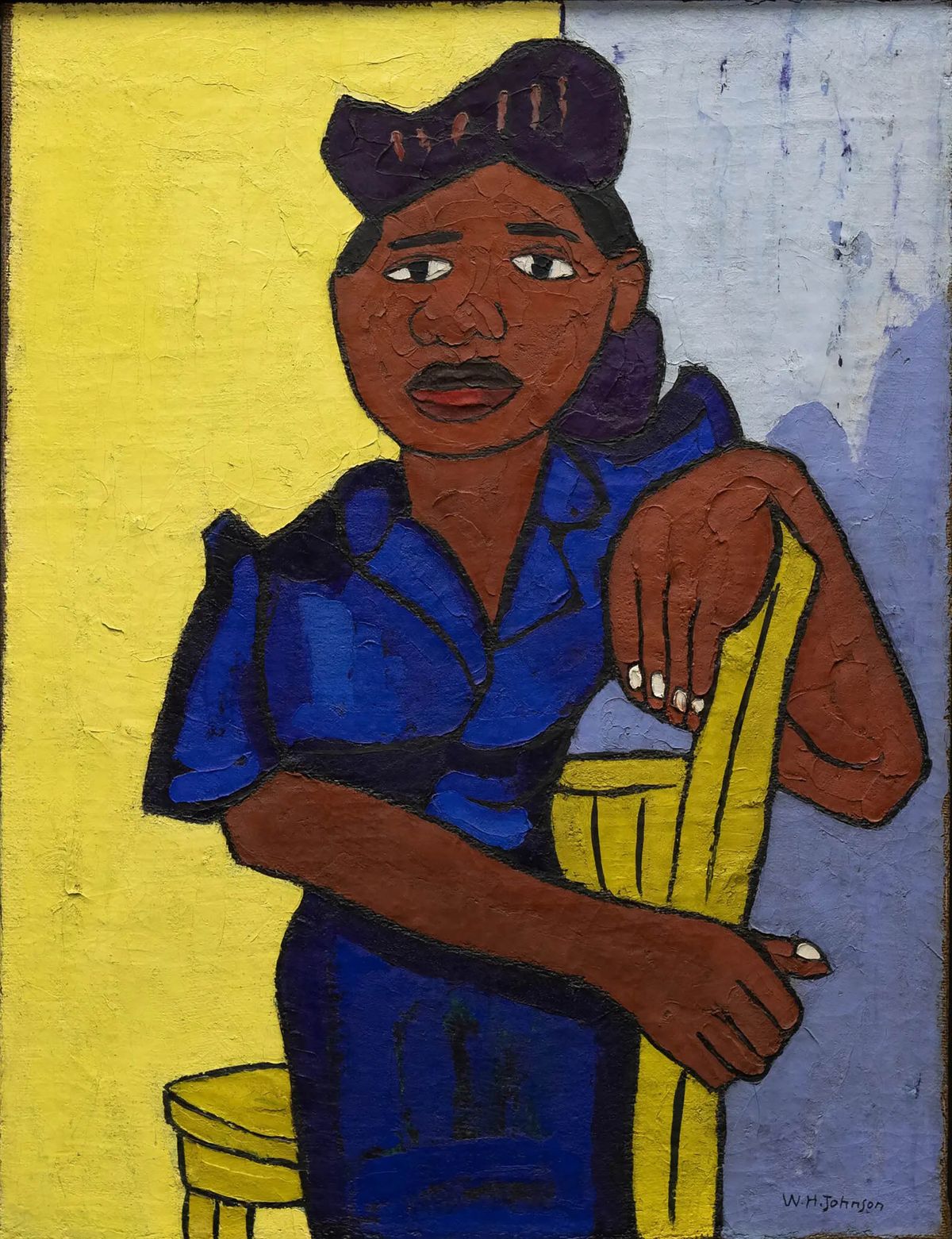This painting depicts a brown-skinned woman with basic, amateurishly rendered features, including a wide face, simple nose, eyes, eyebrows, and lips. She has dark hair styled in an oddly shaped bun or hat-like form, which appears slightly purple. The woman is wearing a dark blue dress with short sleeves and has her white-fingernailed hands interacting with a high-back chair; her right arm grips the back of the chair while her left arm drapes over its top. The background is divided vertically, with about 60% being a medium to light yellow on the left and the remaining 40% a gradient from light blue at the top to darker blue at the bottom, where her shadow is visible. The artist's signature is located in the bottom right corner of the painting. The image suggests a somewhat abstract composition with the chair's seating part obscured behind her legs.